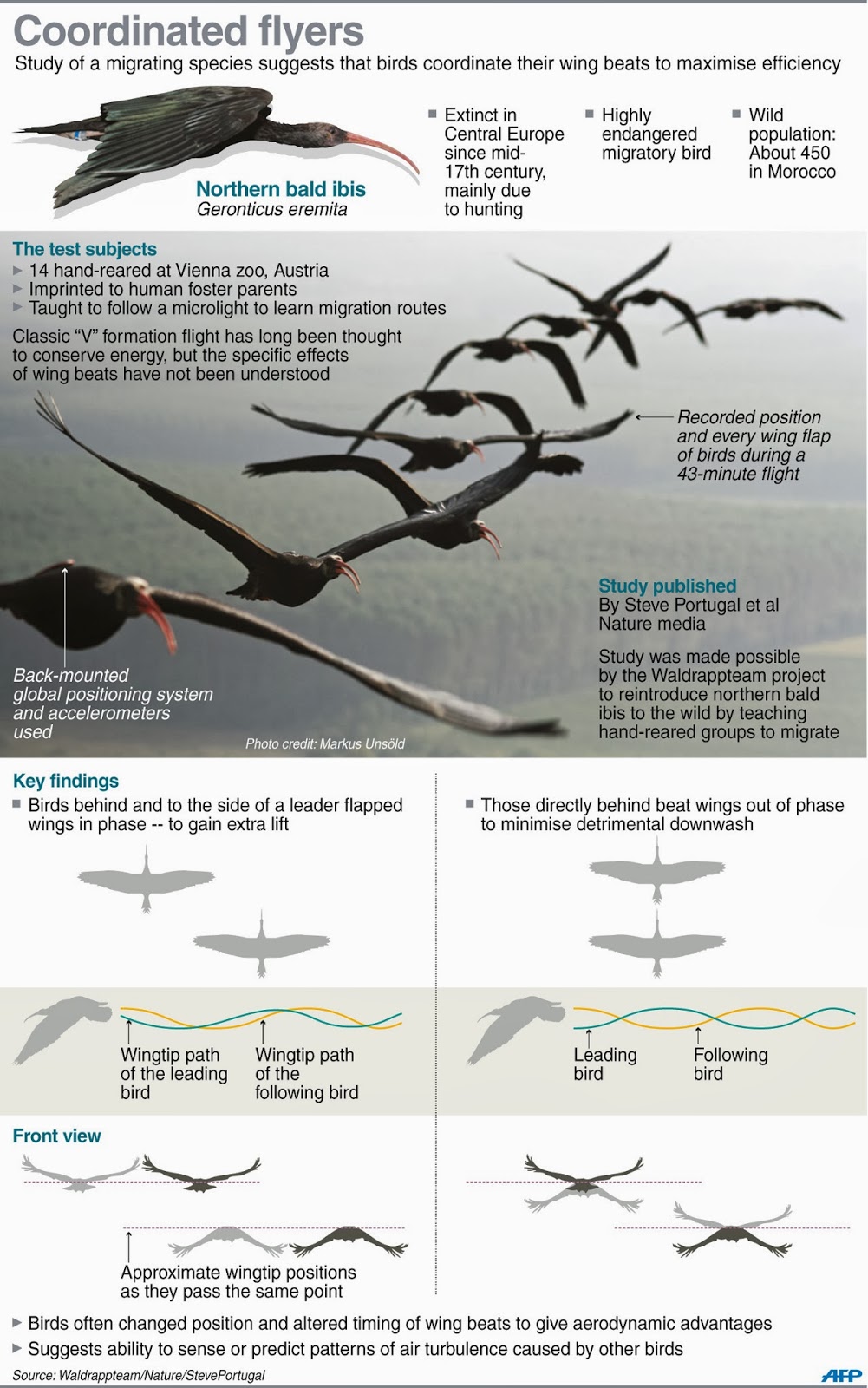The image presents a detailed scientific study on the migratory behaviors of the highly endangered Northern Bald Ibis (Geronticus eremita), extinct in Central Europe since the mid-17th century primarily due to hunting. Set against a white background, the top section features gray text that states, "Coordinated Flyers: Study of a migrating species suggests that birds coordinate their wing beats to maximize efficiency." The main visual element is a formation of Northern Bald Ibises in flight, demonstrating their synchronized wing beats. These ibises, described as black, long-bodied birds with distinctive orange beaks, are shown flying in a V formation, indicating a highly coordinated effort to conserve energy during migration. 

Detailed insights reveal that there are approximately 450 individuals left in the wild, primarily in Morocco. The study evidently involves 14 hand-reared ibises from the Vienna Zoo in Austria, which were imprinted on human foster parents and taught migratory routes by following a microlight aircraft. The lower section of the image includes anatomical diagrams of the birds' wings, with front and reverse views, as well as indicators showing the positions of their wings during a recorded 43-minute flight. Additional graphical elements, such as arrows and wave patterns in green and yellow, highlight the aerodynamic pathways and formations that contribute to their efficient flight. This visual and textual amalgamation comprehensively outlines the methodologies and findings of the bird migration study.